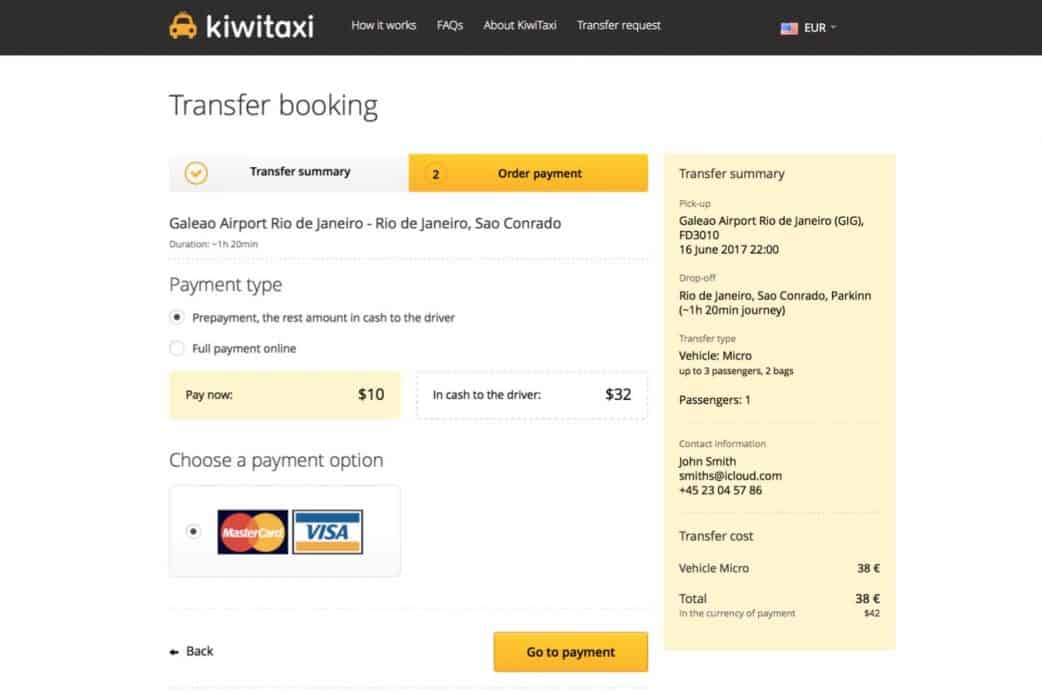**Detailed Image Caption:**

The interface showcases a payment page for Kiwi Taxi. At the top of the screen, there is a black border featuring the Kiwi Taxi logo on the far left - a yellow or orange taxi cab icon with the text "Kiwi Taxi" in white font. Moving right, the menu options are labeled "How it works," "FAQs," and "Transfer Request." Next to these is a currency dropdown marked "EUR," accompanied by a European flag icon.

Below this border, the main body of the page has a white background titled "Transfer Booking." This section is divided into two columns. The left column begins with a segment called "Transfer Summary," marked with a yellow checkmark icon. Immediately below is a highlighted section titled "Order Payment." This section details the transfer specifics: 

- From Galeão Airport, Rio de Janeiro (Galeão Airport) to Rio de Janeiro, Seocondrado.
- Payment options available are prepayment, partial payment (rest in cash to the driver), or full payment online.
- A prompt to pay "Now $10," with the remaining $32 to be paid in cash to the driver.
- Options for selecting a payment method, either MasterCard or Visa, followed by a "Back" button and a prominent yellow "Go to Payment" button.

The right column provides a "Transfer Summary" for clearer details:
- Pickup: Galeão Airport, Rio de Janeiro.
- Flight Number: FD3010.
- Date and Time: 16 June 2017, 22:00.
- Drop Off: Rio de Janeiro, Seocondrado.
- Duration: 1 hour and 20 minutes.
- Vehicle: Micro (suitable for up to 3 passengers and 2 bags).
- Passengers: 1.
- Contact Information: John Smith (email: smiths@icloud.com, phone: 4523045786).
- Transfer Cost: €38, with the total amount in another currency being $42.

This detailed interface provides comprehensive booking information for a taxi transfer, ensuring all essential details are clearly presented to the user.